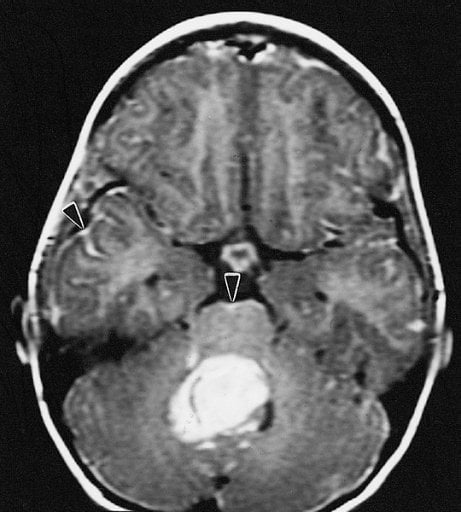This image showcases a detailed CT scan of a brain viewed from above against a solid black background. The outer edges of the skull are distinctly outlined in white. Inside the skull, various regions of the brain are depicted in gray, white, and black tones. Notably, there are distinct black arrows within the scan: one arrow on the left points downward to a brain section, and another in the center directs attention to the bottom section of the brain, which features a prominent light spot. Additionally, a white dot can be seen in the center of the brain. Around the ears, there are faint whitish outlines, adding to the intricate details of this radiographic image.